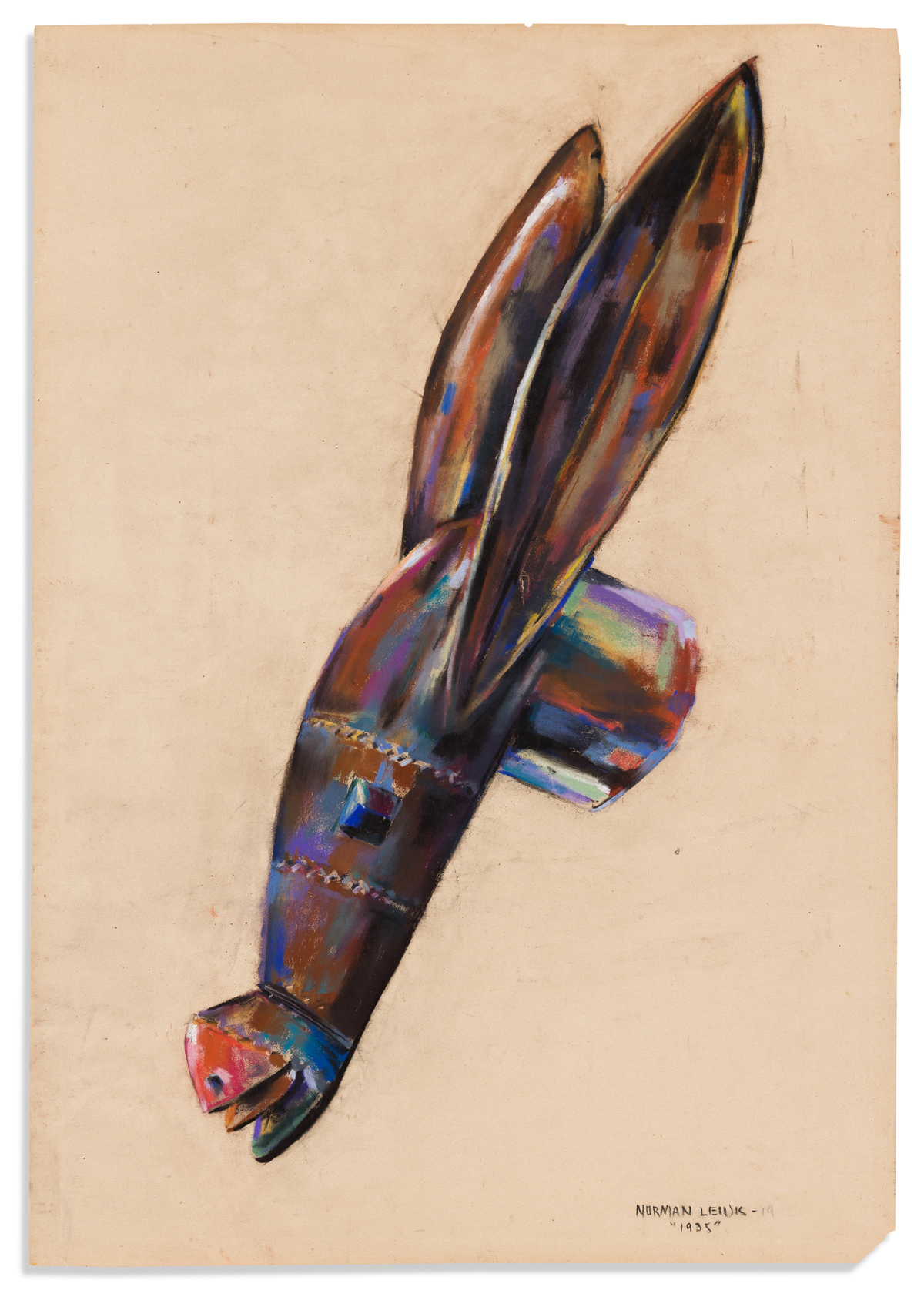The image is an art print on light brown paper, featuring a surreal, abstract portrayal of a long, slender donkey's head. The artwork is signed in the bottom right corner with "Norman Luke, 1935," and the corner of the paper is slightly folded. The head, facing to the right, has a rust-colored forehead and long ears, reminiscent of rabbit ears, with one ear being rust-colored with a white highlight and the other a darker shade. The nose is red, the mouth is small, and the eye, strikingly blue like a jewel, is set on the side. Above and below the head are lines that enhance its abstract nature. The neck is a blend of blue, white, black, reddish, purplish, and green hues, giving it a metallic and shiny appearance. The overall piece combines elements of abstraction and surrealism, depicting an artistic representation that blends the features of a donkey, a horse, or perhaps a bird or insect diving.